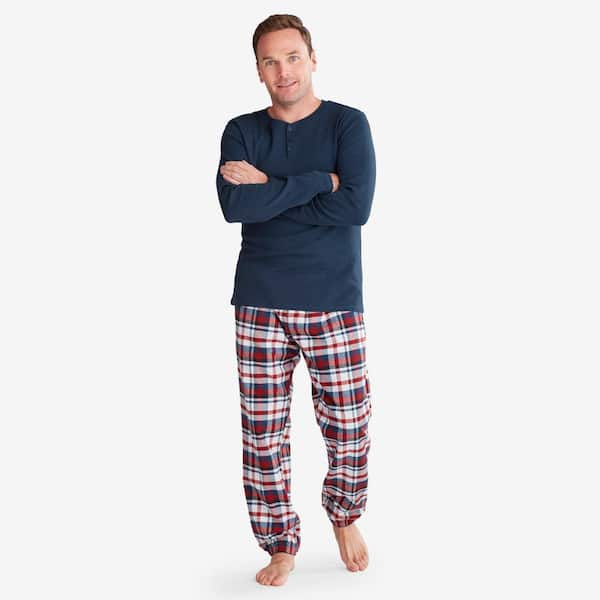This image depicts a generically attractive white male, likely in his late 20s to early 30s, posing against a stark white background often used in advertisement photos. The man stands barefoot, comfortably dressed in a navy blue, long-sleeved thermal Henley shirt with buttons at the neckline and a pair of loose, flannel pajama bottoms featuring red, blue, and white striped plaid. He has short brown hair combed over to the left and blue eyes. His face is adorned with stubble and thin eyebrows, and he sports a slight, peaceful grin while looking slightly to the left of the camera. Standing at a height that almost touches both the top and bottom edges of the frame, he exudes a relaxed and calm demeanor with his arms casually crossed over his chest. His left foot rests flat on the ground, while his right toes are pointed and just touching the ground, enhancing the overall sense of coziness and ease.